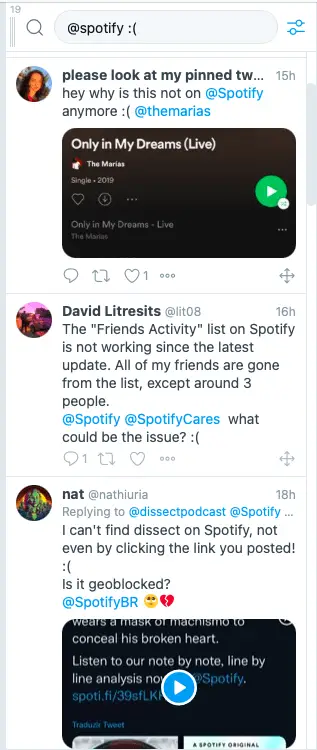Here's a polished and detailed caption for the image:

---

The image depicts a screenshot of a Twitter thread where users are voicing their concerns and issues with the Spotify platform. At the top of the interface, the search bar contains a sad face emoji, and there is a settings-like toggle switch on the right side.

In the first tweet, a woman with long dark hair, using the handle @Mariahs, expresses her frustration about a missing song. Her tweet reads: "Please look at my pinned tweet, why is this not on @Spotify anymore?" She has attached a note that says "Only in my dreams" by The Marías, indicating her desire to understand why the song has been removed from the platform. Her tweet has garnered one like.

The second tweet in the thread is from a user named David Letresic, who reports an issue with the Friends Activity feature on Spotify. He writes: "The friends activity list on Spotify is not working since the latest update. All of my friends are gone from the list except around three people. @Spotify @SpotifyCares, what could be the issue?"

Following that, there's a reply from another user, Nat, mentioning a different problem. She states: "I can't find Dissect on Spotify, not even by clicking on the link you posted. Is it geo-blocked? @SpotifyBR" along with a screenshot of her issue.

This Twitter thread highlights various user frustrations regarding missing songs, issues with updates, and potential regional content restrictions on Spotify.

---